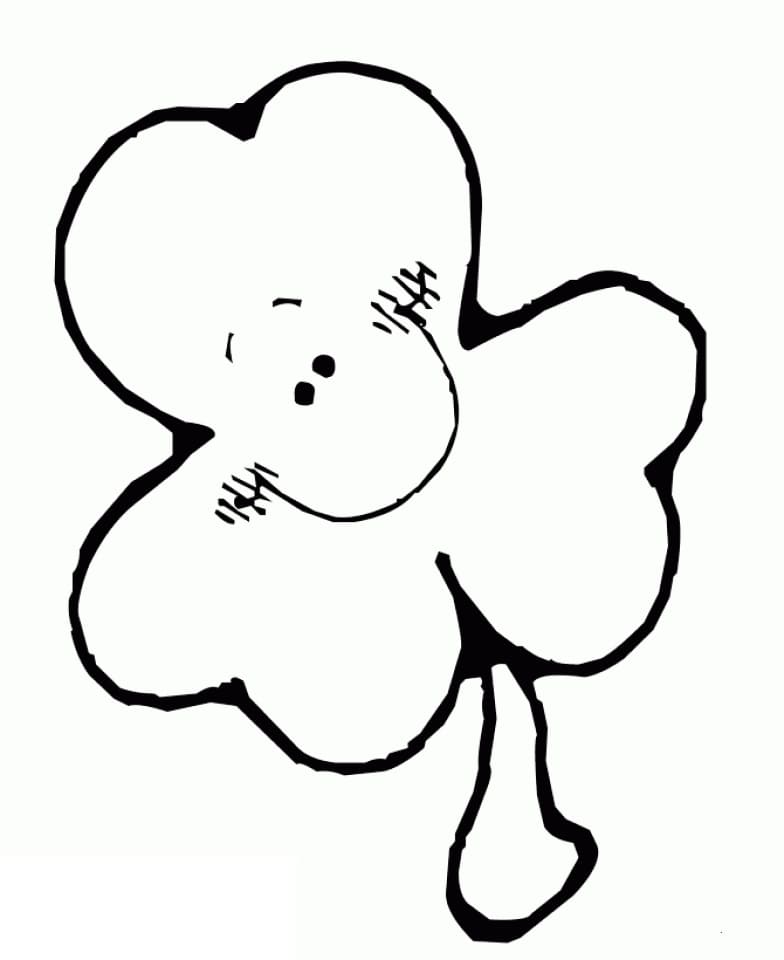This image features a simplistic, cartoon-style drawing of a three-leaf clover, rendered in a black outline against an eggshell white background. The clover, positioned diagonally in the center, exudes a charming, childlike quality with its rough, jagged edges. Each leaf resembles the top half of a heart, collectively forming a whimsical shamrock shape. In the middle of the clover is an expressive smiling face with two round eyes and small black eyebrows arched above. The wide, semicircular smile is flanked by diagonal lines that add to the cheerful expression by suggesting rosy, chubby cheeks. Below the clover’s leaves, a curved stem extends downward, completing the playful and endearing design. The entire drawing, reminiscent of something from a children's coloring book, is devoid of any color or text, leaving only the stark contrast of black and white.